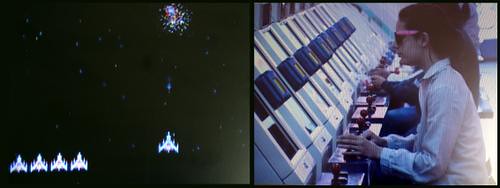The image is a landscape-oriented photograph with a thin black border, divided into two sections. On the left side, there's a pixelated, computer graphic screen reminiscent of a Space Invader game. This screen features a night sky-like backdrop with what appears to be a firework or explosion in the top right corner. At the bottom left are four triangular spaceship shapes, likely representing game characters or lives, and another spaceship slightly higher up towards the center, apparently shooting at the exploding object. In the right section of the picture, there is a photograph showing a woman with black hair pulled back, wearing pink-rimmed sunglasses and a white collared jacket. She is intently playing a video game at a console, which is slightly tilted to the left. In the background, another person, presumably a girl in blue jeans with dark hair, is partially visible. The setup includes joysticks and red-buttoned controls, suggesting an arcade environment, with multiple arcade machines lined up.